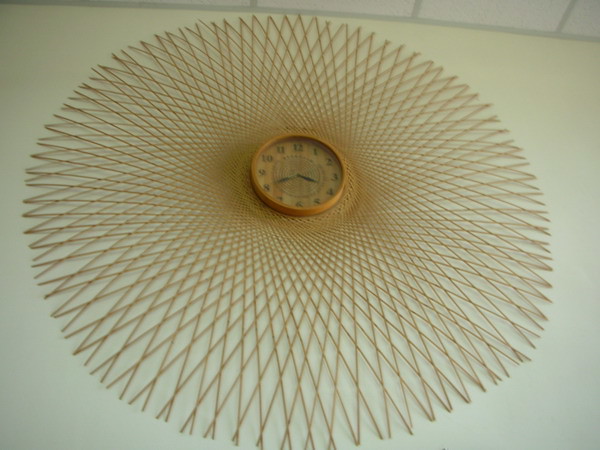The photograph features an analog clock mounted on a wall, which is a uniform off-white or ivory color. The upper portion of the image reveals some white ceiling tiles, divided into squares by gray lines. Centrally placed, the clock itself has a circular wooden frame with a gold-hued rim. The worn face of the clock displays the numbers 1 through 12, and the time reads approximately 3:40. A unique geometric pattern radiates from the center of the clock, comprising numerous gold lines that intersect to form a diamond pattern. This intricate design begins with smaller diamonds close to the center and expands into larger ones as it fans outward, producing a sunburst or web-like effect.